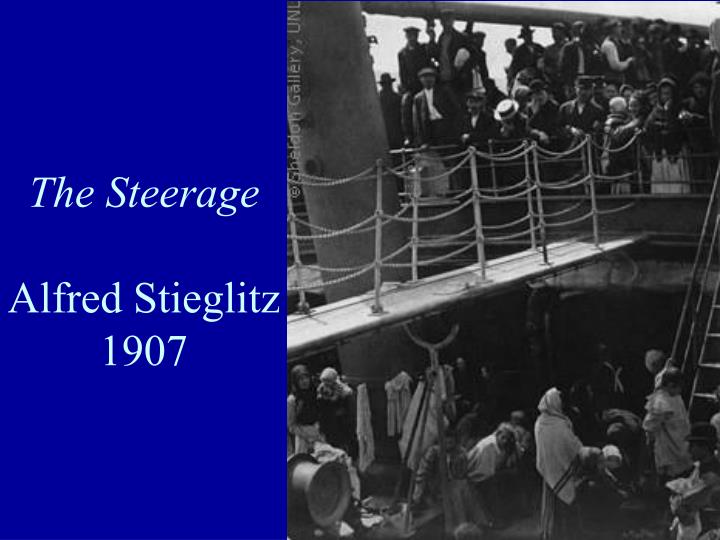The image is a horizontal rectangular slide featuring a black and white photograph by Alfred Stieglitz titled "The Steerage," taken in 1907. On the left third of the image, a solid blue background in white Times New Roman font highlights the title "The Steerage," the photographer's name, "Alfred Stieglitz," and the year "1907." The photograph occupies the right two-thirds of the slide and depicts a scene on a ship with a clear class divide. The lower level, referred to as the steerage, shows poorly dressed individuals, some with hanging clothes on makeshift lines, suggesting their lower economic status. They appear disheveled and down on their luck. A chain-link barrier separates them from an upper level where better-dressed individuals in hats and formal attire are gathered, indicating their higher social class. The overall scene is crowded and bustling, capturing a poignant moment in early 20th-century travel.